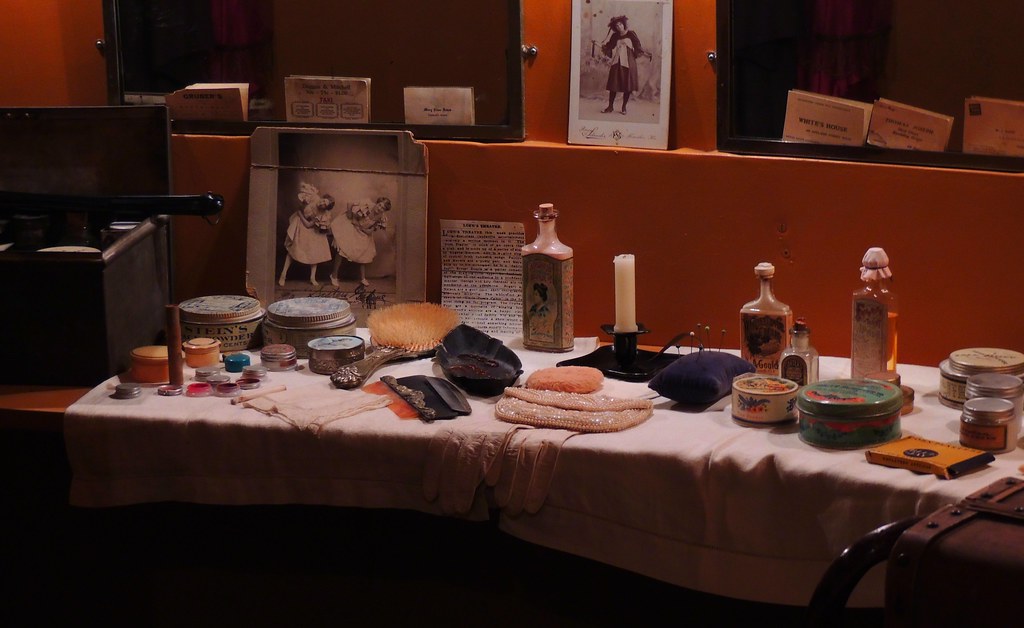This image depicts a vintage-themed dressing table set against an orange backdrop. The background features an orange wall with a thin ledge, where two black-framed mirrors rest, each holding three business cards at their base. Positioned between the mirrors, a black-and-white Polaroid picture adds to the nostalgic ambiance. Below, the table is draped in a white cloth and showcases a collection of antique and beauty items. The left side of the table holds an aged black-and-white photograph of two women, possibly from the early 1900s, dressed in costume-like skirts, hinting at a vaudeville or old theatre theme.

The tabletop displays an assortment of vintage objects, including an old-fashioned silver-handled hairbrush, a white candle in a black base, and various containers of beauty powders and makeup tins adorned with intricate designs. Antique-looking bottles, candle holders, and perfume bottles complement the scene, alongside makeup brushes and sponges, creating an air of bygone elegance. The room, dimly lit with an overhead light emphasizing the table, is cloaked in deep mahogany and dark red shades that add to its shadowy, almost museum-like display ambiance.